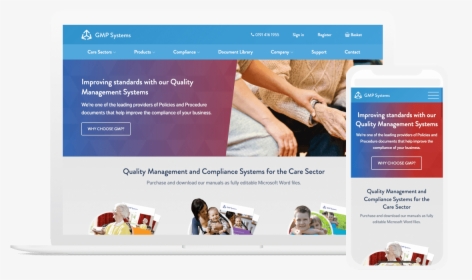The screenshot displays the homepage of the GMP Systems website, characterized by two horizontally-aligned blue bars at the top. The upper bar is a darker blue than the one below it, and both feature white text. 

Beneath these bars is a visually striking graphic. The upper portion of this graphic shows a photograph, starting from the left with a deep blue color that gradates into purple. The photo captures a close-up view of two individuals' laps. The person on the left has their hand resting on the wrist of the individual to the right, while their other arm is draped across their leg.

The section below this graphic is light gray and prominently displays the phrase "Quality management and compliance systems for the care sector." At the bottom of this section, there are three smaller images: on the left is an iconographic representation of a lady, in the middle is a picture of a lady and a baby, and on the right appears to be an image of a child.

In the bottom right corner of the screenshot is an inset image of a cell phone, which displays the same webpage.